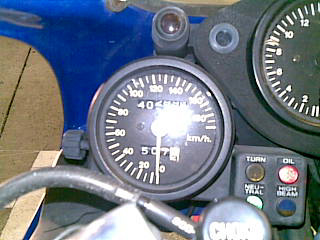This small, low-quality, and slightly blurry square photograph captures a close-up view of a motorcycle's dashboard. Dominating the center of the image is a standard speedometer encased in a gray plastic base with a clear plastic cover. The speedometer dial ranges from 0 to 200, and the needle is pointing to 0. A large, white light reflection is prominently visible on the clear cover. Below the speedometer, to the left, part of the motorcycle's handlebar is visible. To the right of the speedometer is a small gray plastic box featuring four buttons: a red button on the top right, next to a white button, with a blue button directly below it, and another white button underneath the blue one. Above the speedometer, partially visible due to the framing of the photograph, is another gauge with a round face set within a black oval. The gauge has a black background with white markings, but only half of it is visible in the image.